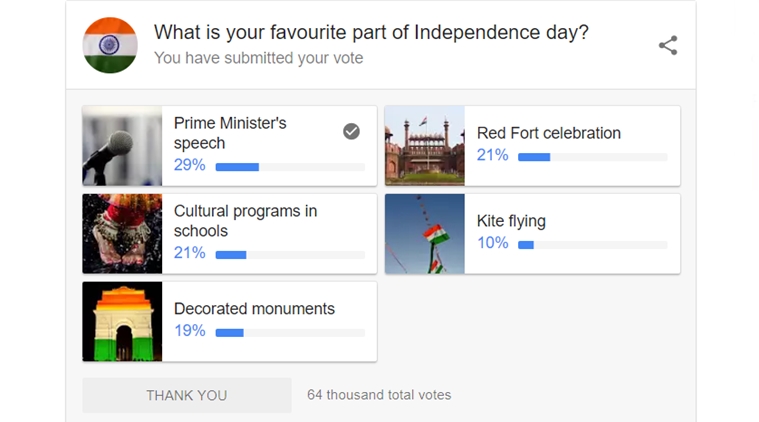This image is a cropped screenshot of a website page. The top section features a white rectangular header. On the far left of the header, there is a circular icon displaying the Indian flag, which consists of an orange stripe on top, a white stripe in the middle with a blue Ashoka Chakra, and a green stripe at the bottom.

In the center of the header, a large black text reads, “What is your favorite part of Independence Day?” Below this, in light gray text, is the message, “You have submitted your vote.” On the far right of the header, there's a dark gray share icon, shaped like three connected circles forming a triangle pointing left, with two gray lines branching out from the center circle to the other two.

Beneath the header, a thin light gray line separates the header from the body of the page, which has a light gray background. The main content displays five tiles. Each tile consists of a square photograph on the left and a white rectangular section to the right. 

In each white rectangle, there is a line of black text at the top left, a blue number at the bottom left, and a corresponding progress bar to the right of the number. The progress bar is light gray with a blue fill indicating progress. The tiles are arranged in two rows, with two tiles on the top row and three on the bottom row, followed by an area of negative space:

1. Prime Minister's Speech
2. Red Fort Celebration
3. Cultural Programs in Schools
4. Kite Flying
5. Decorated Monuments

At the bottom, beneath the last tile, there is a light gray box with dark gray all-caps text that says “THANK YOU.”